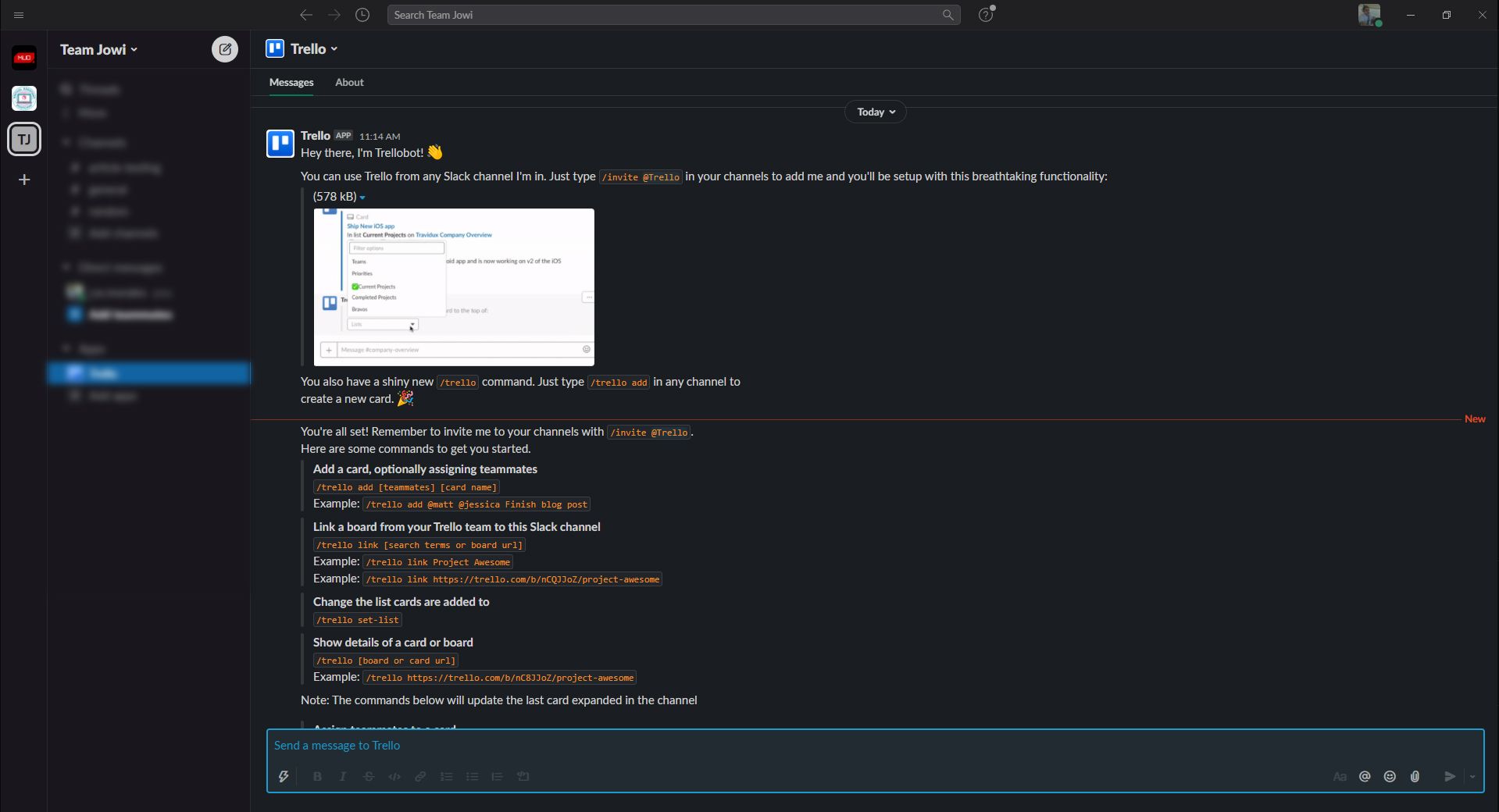A screenshot displays an interface with a black background at the top. Below the black header is a gray search bar labeled "search team Jowl." Under the search bar, there are tabs with labels including "Trello," "Messages," and "About." The interface also indicates that the current message is listed under "Today."

In the main section of the interface, a prominent blue box is displayed. Inside this blue box are two smaller white boxes. The text within the blue box reads: 

"Trello
Hey there, I'm Trello Bot. You can use Trello from any Slack channel I'm in. Just type /invite @Trello in your channel to add me and you'll be set up with this breathtaking functionality."

Beneath the blue box, there is another box containing text that is not fully visible. Below this hidden text, more instructions are provided in a conversational tone:

"You also have a shiny new Trello command. Just type /trello add in any channel to create a new card.

You're all set! Remember to invite me to your channel with /invite @Trello. Here are some commands to get you started:
- Add a card, optionally assigning teammates: /trello add [teammates] [card name]"

This descriptive caption vividly captures the content and appearance of the interface, enabling an accurate understanding of the Trello Bot's functionality and setup instructions within Slack.